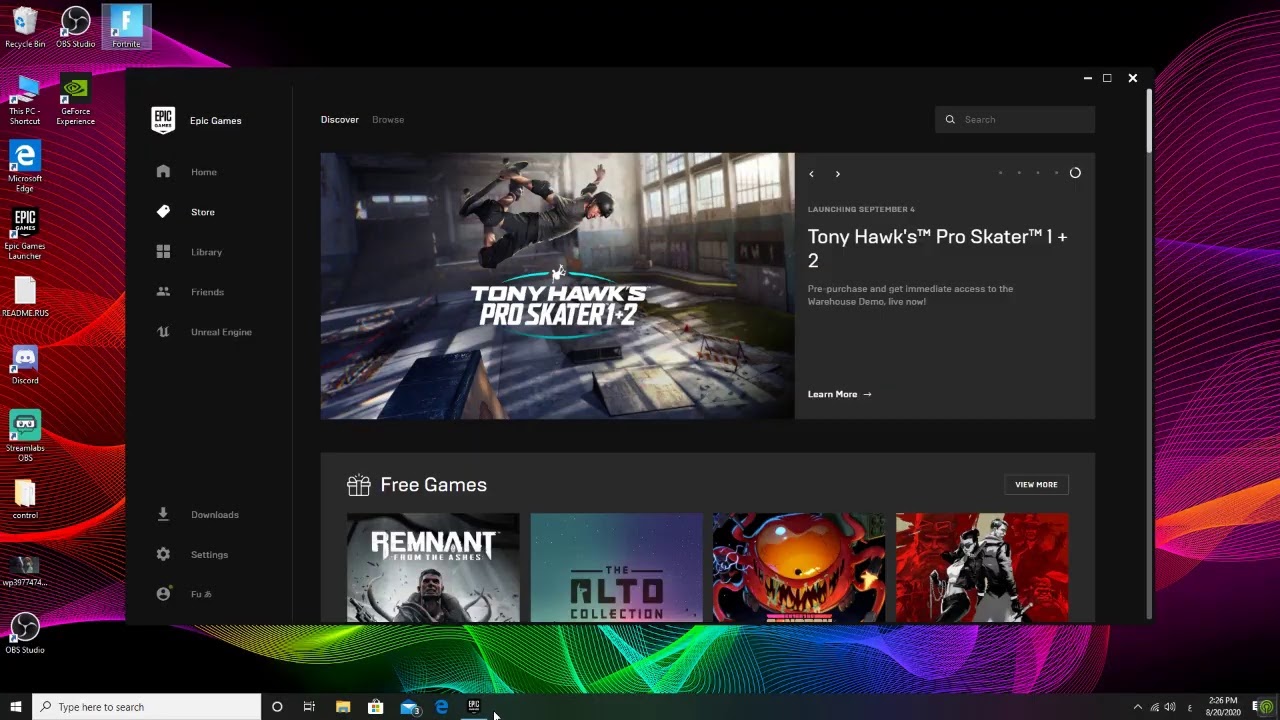The image appears to be a vibrant screenshot from a video game interface. The background is a mesmerizing swirl of varied colors including green, red, purple, blue, and light pink. The screen displays vertically aligned icons on the left and another set of icons on a blue bar descending on the right side.

Prominently, there’s an area dedicated to Tony Hawk's Pro Skater 2 showcasing a sketch of Tony Hawk mid-air, gripping his skateboard with a green circular landing spot beneath him. The title "Tony Hawk's Pro Skater 1 and 2" is displayed in a gray section to the right. Below this, there's a section labeled "Free Games" featuring titles like "Remnant" and "Alto." Additionally, the interface includes images presumably from other video games: a massive spider-like creature and a modern-day robot.